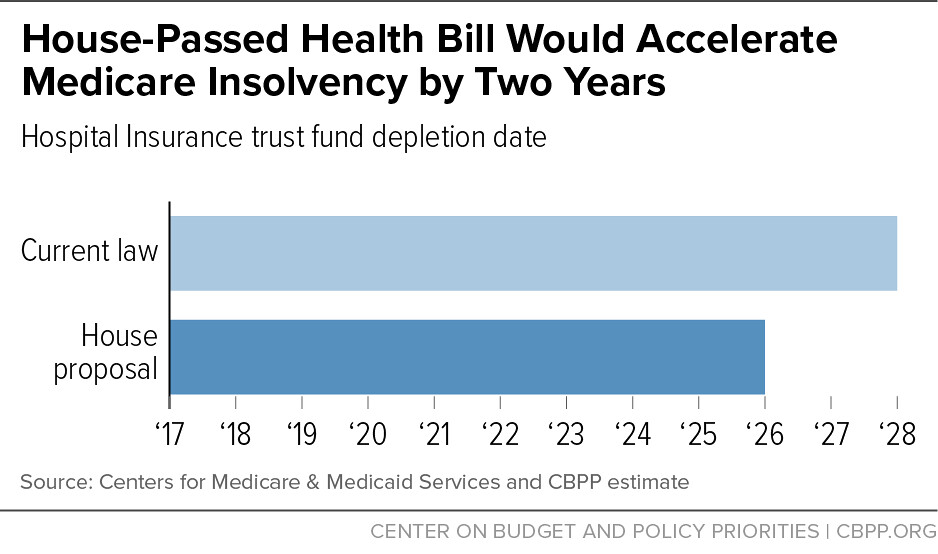The image is an infographic depicting the impact of a House-passed health bill on Medicare insolvency. At the top, the title reads: "House Passed Health Bill Would Accelerate Medicare Insolvency by Two Years." This is followed by a subtitle in black, stating: "Hospital Insurance Trust Fund Depletion Date." Two horizontal bars are used to illustrate the data, with "Current Law" on the left side represented by a light blue bar extending until the year 2028, indicating the projected depletion date. Below it, a darker blue bar represents the "House Proposal," which shortens the depletion timeline to 2026. Along the bottom of the chart is a scale ranging from the years 2017 to 2028. The source of the data is attributed to the Centers for Medicare & Medicaid Services and CBPP estimates, with a note at the bottom reading: "Center on Budget and Policy Priorities CBPP.org."